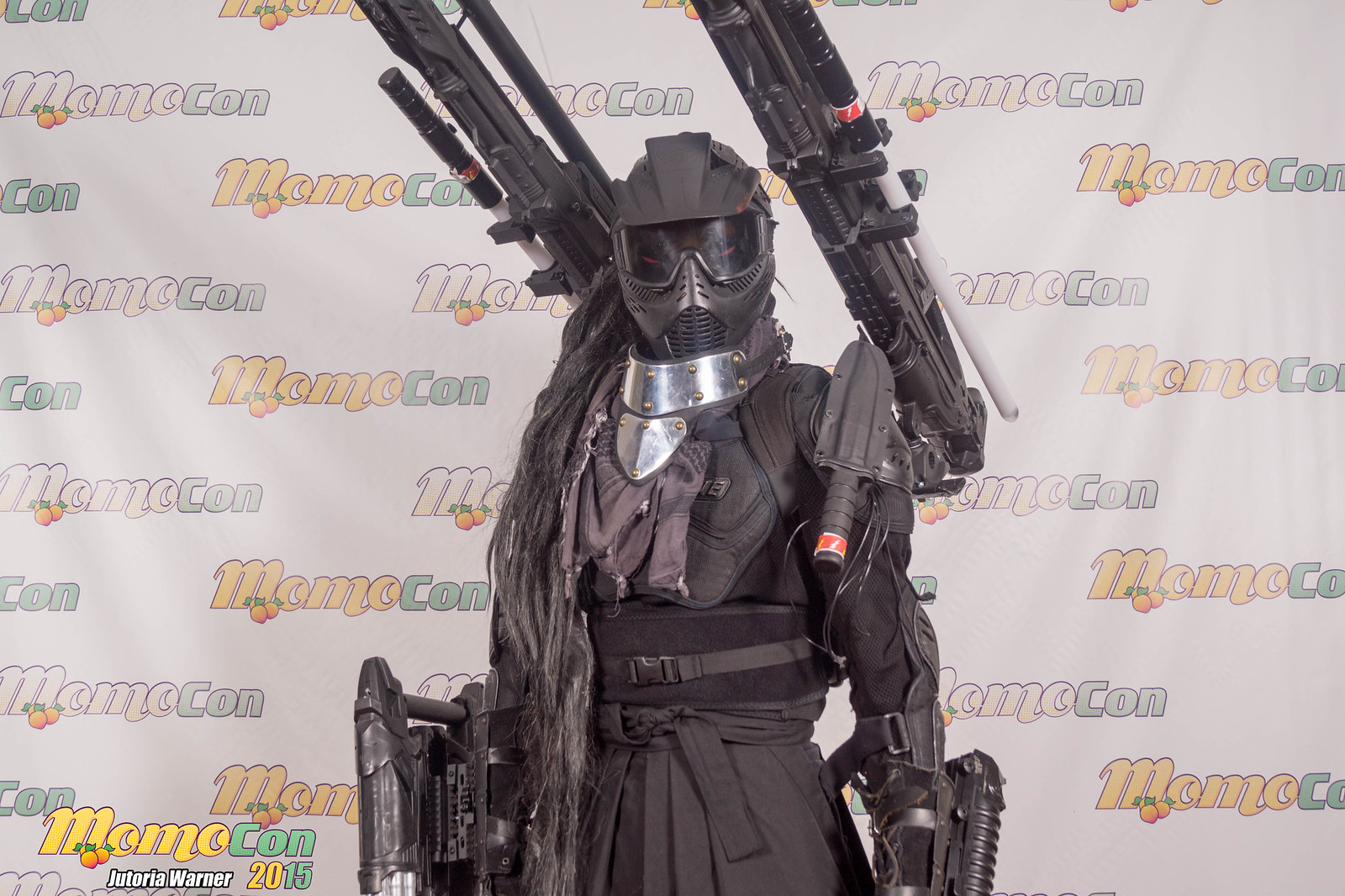This landscape-oriented color photograph captures a highly detailed and realistic depiction of a cosplayer at MomoCon 2015. The subject, dressed as a dark warrior ready for an apocalyptic battle, stands in front of a white banner adorned with the MomoCon logo—'MOMO' in yellow and 'CON' in green letters. The bottom left corner of the banner features the text "Deuteria Warner, 2015."

The cosplayer, possibly a female figure, is clad in an elaborate and high-quality black military-style uniform. Their samurai-like attire includes an akama and an obi, complemented by dark armor resembling a bulletproof vest. They wear a menacing paintball mask with dark goggles, obscuring their face, and a metallic neck covering. Long, dark, dreadlocks or hair extensions cascade down the left side of their front.

The striking warrior is heavily armed, wielding large machine guns in both hands and shouldering two rifles, while additional heavy machine guns are strapped to their back. The overall appearance evokes a blend of samurai and futuristic warrior aesthetics, resulting in a captivating and fierce visual presentation.